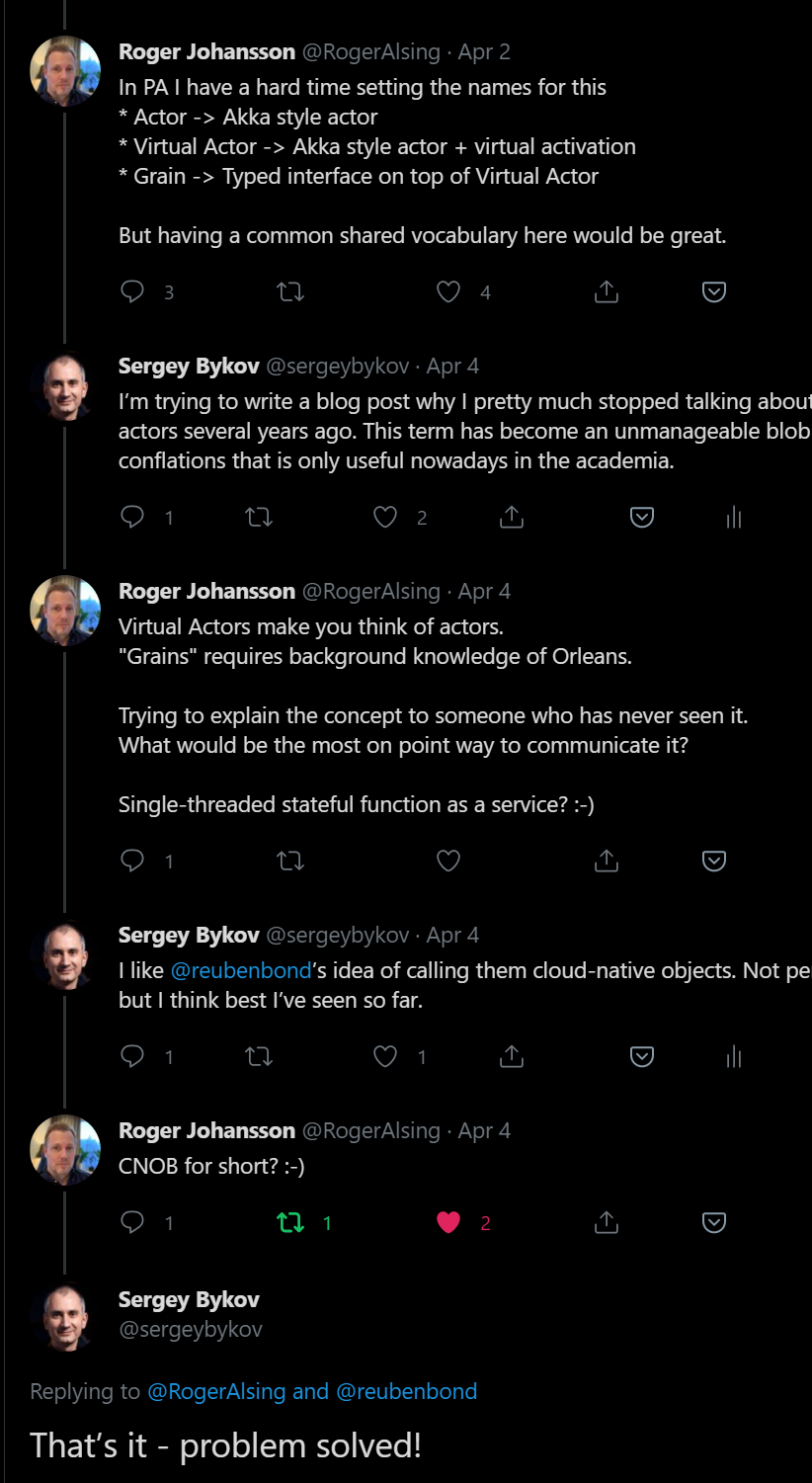**Screenshot of a Technical Conversation:**

The image is a screenshot likely taken from a smartphone, featuring a conversation with a black background and white text. At the top of the image, there's a profile picture of a white man inside a circle, identified as Roger Johansson. 

Roger starts the conversation: "In PA, I have a hard time setting the names for this. Actor, aka-style actor, virtual actor, aka-style actor plus virtual activation, grain-type interface on top of virtual actor. But having a common shared vocabulary here would be great."

Following Roger, another participant appears, whose profile picture is also that of a white man, named Sergey Bykov. Sergey responds: "I'm trying to write a blog post about why I pretty much stopped talking about several actors several years ago. This term has become an unmanageable blob conflation that is only useful nowadays in academia."

Roger then comments: "Virtual actors make you think of actors. Grains requires background knowledge of Orleans. Trying to explain the concept to someone who has never seen it, what would be the most on-point way to communicate it? Single-threaded stateful function as a service."

The conversation continues with a few more exchanges between the participants, delving further into the terminologies and concepts. At the bottom right of the image, a final remark indicates the resolution of the discussion: "That's it, problem solved."